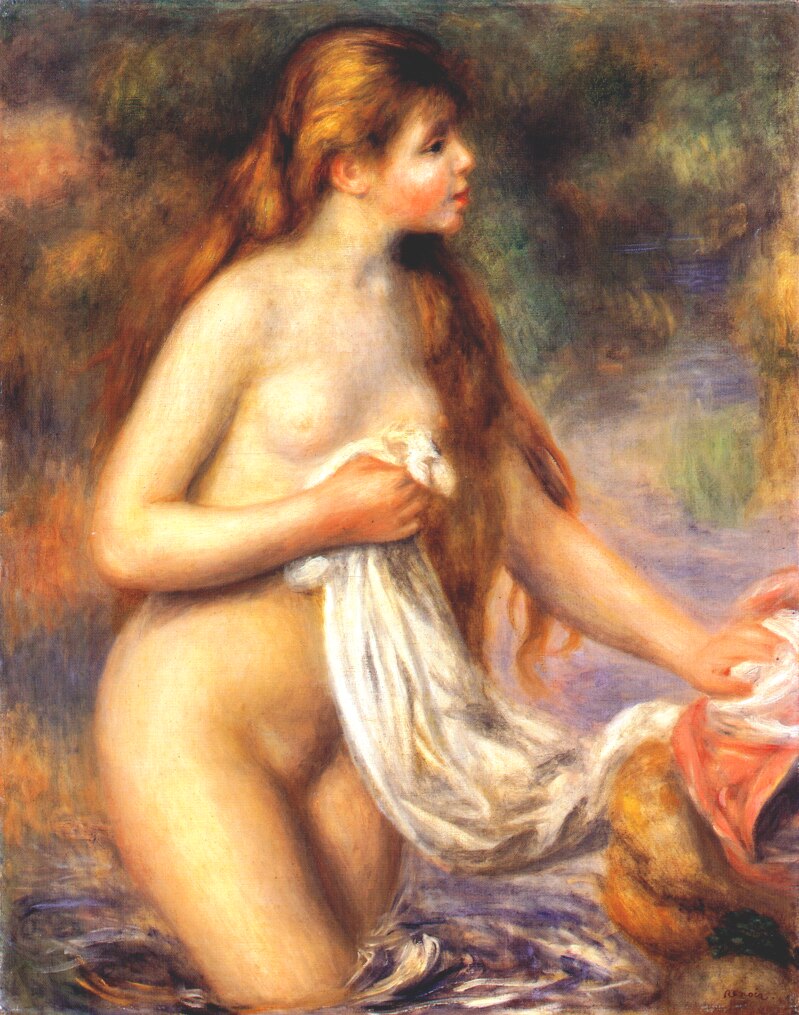This detailed Renaissance-style painting features a nude woman emerging from a stream or lake. Her long, reddish-brown hair cascades down to her hips, and she holds a piece of white fabric, possibly a towel, in both hands. She has fair, peach-toned skin with subtle red and yellow undertones, and a gentle, almost shy smile graces her red lips and rosy cheeks. The water around her legs is a rich, dark blue, interspersed with swirling whites and reflective hints of yellow and peach. The background, softly blurred and not heavily detailed, suggests a natural setting with greens and browns indicative of foliage and trees. The overall painting has a soft, glowing quality with gentle edges, making the woman the clear focal point as she looks to her right, bathed in the delicate play of light and water.